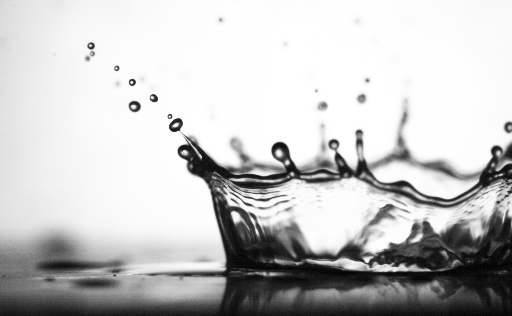In this high-speed, black-and-white photograph, we're presented with an extreme close-up view of a liquid surface, possibly water, which captures the dramatic aftermath of an object being dropped into it. The image is meticulously detailed, showing a dynamic splash that extends from nearly the bottom to halfway up the frame. This splash forms a striking, crown-like shape with numerous spikes, each adorned with tiny water droplets or bubbles that haven't yet separated. Some of these droplets are seen in mid-flight, suspended in the white background and scattered almost to the top left corner. The overall composition highlights the clarity and beauty of the liquid's reaction, making the droplets appear almost like delicate tendrils reaching into the air.